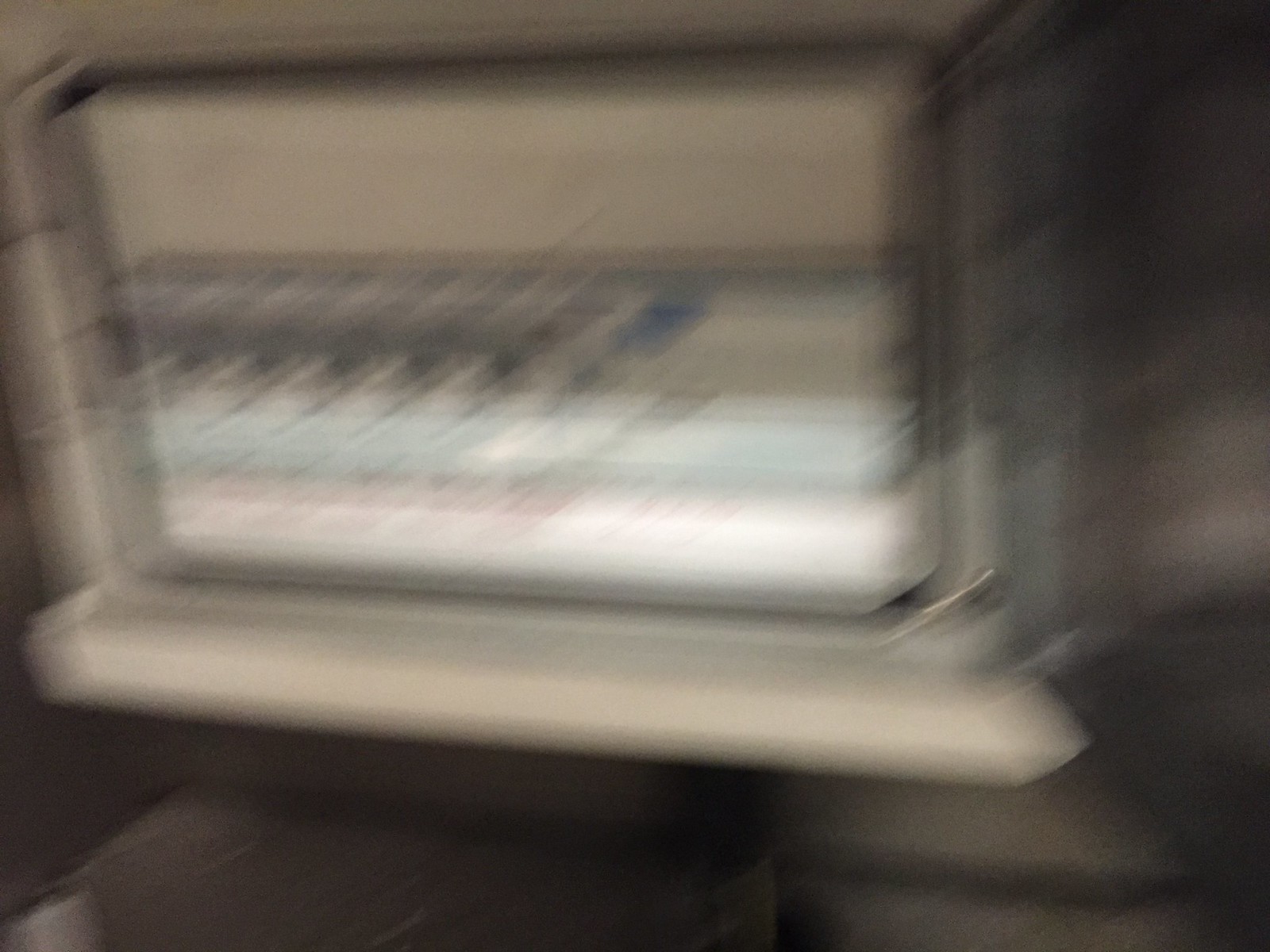The image displays an extremely blurry object that is difficult to identify. The backdrop is composed of various shades of gray, ranging from medium gray to darker tones, and includes small, horizontal rectangular shapes. The central object, reminiscent in shape to a microwave or air conditioner, is a large rectangular cube that appears to run horizontally. Its front features a prominent face with a distinctive white bar below it, which contributes depth to the right side of the object.

The upper quarter of this front panel is a solid grayish-white color. Below this section, there is a series of lines: a light gray line, followed by diagonal lines in darker gray and blue. These are intersected by a horizontal light blue line and a white horizontal line, adding a complex, layered appearance to the panel. The overall composition is defined by its abstract and enigmatic qualities, amplified by the blurriness of the image.